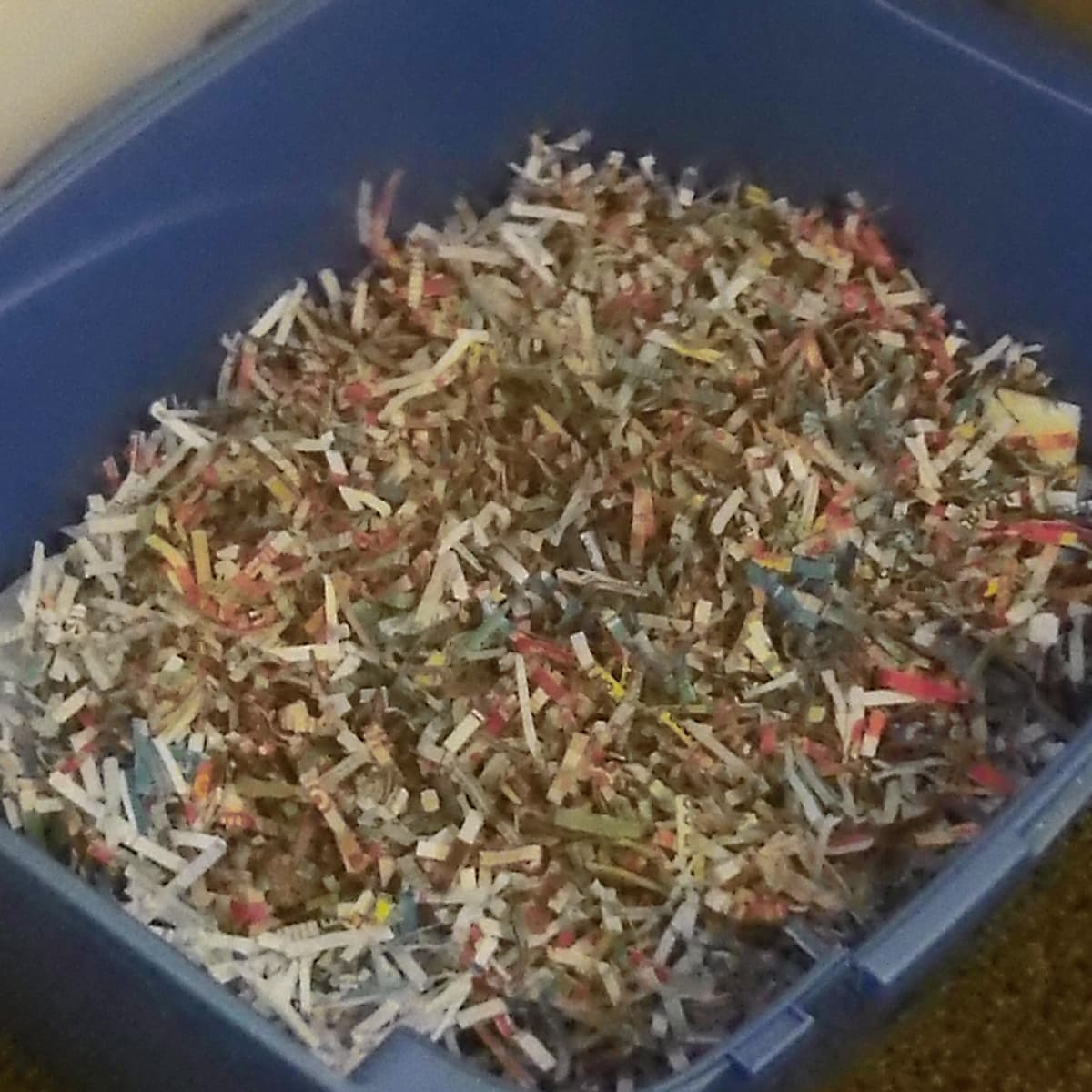This color photograph captures the interior of a blue plastic bin filled with finely shredded paper, located at the bottom segment of a paper shredder. The shredded contents, which appear to be strips from various documents, are brightly colored, including white, yellow, gold, silver, pink, red, and blue. The bin is positioned against a somewhat off-white or light gray wall in the top left corner, while the bottom right corner of the image reveals a portion of a brown rug, suggesting it's part of a room's floor. The container, which appears quite deep and halfway filled, hints at the mundane process of paper shredding turning vibrant through the colorful mix of shredded magazine pages. The photograph exudes a slightly washed-out, nostalgic feel reminiscent of early 90s home photography.